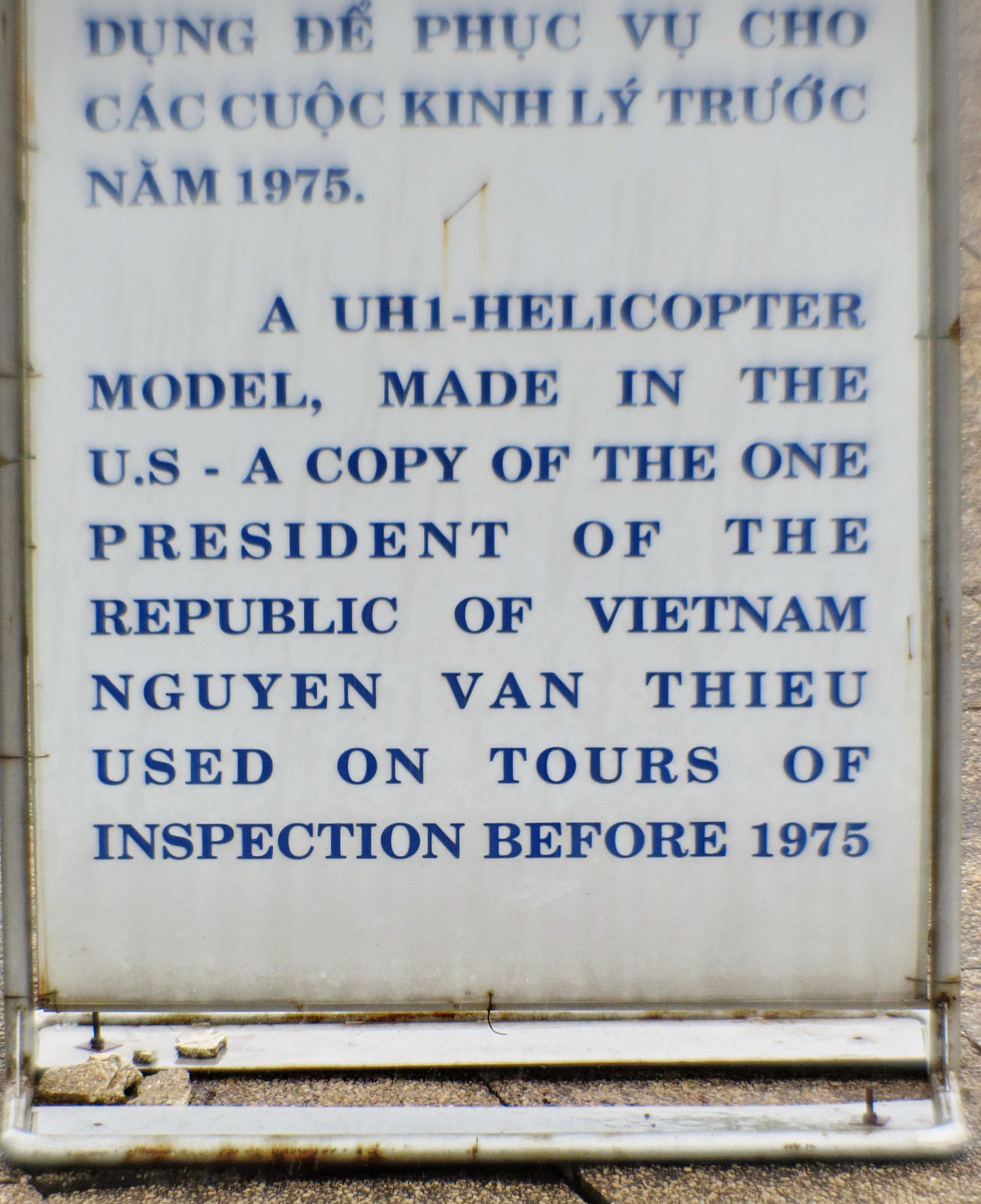The photograph showcases a freestanding metal sign with a white background and dark blue, capitalized text. Situated outdoors on a grayish-brown concrete surface, the sign is placed centrally within the image, which appears to be zoomed in, making the periphery blurry and soft. The sign features both Vietnamese and English text. The Vietnamese text is at the top, followed by English text that narrates the historical significance. It mentions a UH-1 helicopter model made in the USA, which replicates one used by the President of the Republic of Vietnam for inspection tours before 1975. This likely indicates that the image was taken at a historical site related to the Vietnam War.